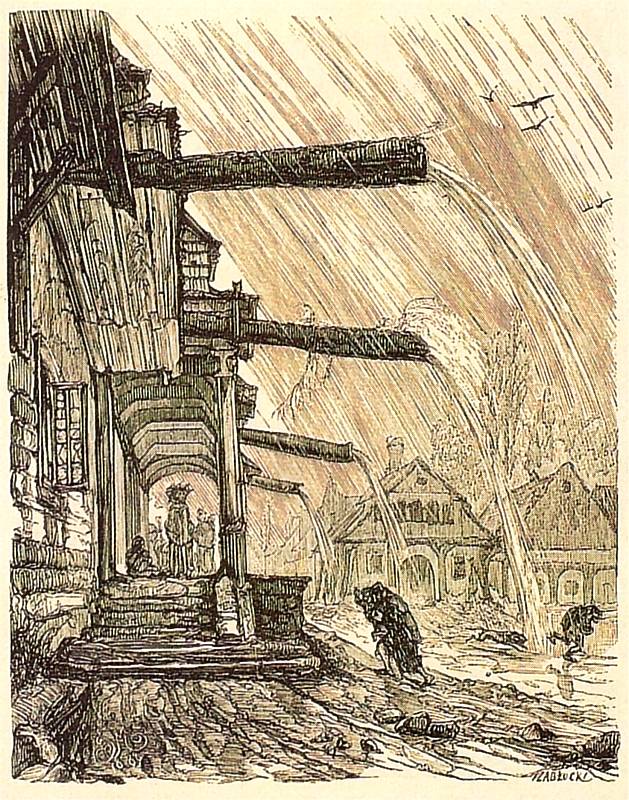This detailed black-and-white woodcut by John Matejko, titled "Wooden Houses in Vishnesh in the Rain" and created in 1863, depicts a small town engulfed in a significant rainstorm. The image, oriented in portrait, showcases the side of a formidable, wooden building on the left, which appears to be a saloon or fortress, with four large water spouts extending at least eight feet from the roof, pouring water onto the road below. Under the pouring rain, two figures are seen hunching down and moving quickly towards the building, seeking refuge under the covered porch, where several people are already standing. The porch is accessible via a large stairway. The lower right corner features houses, and another individual is bent over, running towards shelter. Above, the sky is animated with streaks of orange and four seagulls flying overhead. The overall style of the piece reflects Romanticism, capturing the dramatic and tumultuous atmosphere of the storm.